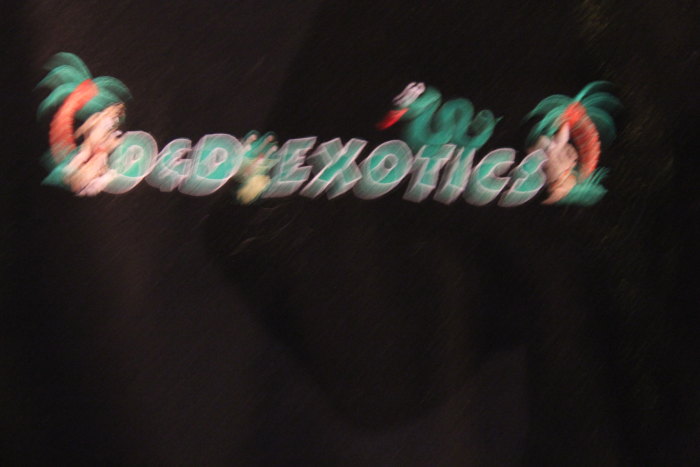The image features a black background adorned with a vibrant and exotic scene. On the top left, there is a palm tree with a distinctive red center and lush green leaves extending to both sides. Dominating the center of the image is a dog with brown fur, a red collar, and large expressive ears. This dog is seated next to a decorative pot labeled "exotics" in elegant letters. Just above the word "exotics," a snake is depicted curling gracefully, its red tongue flickering outwards. On the far right side of the image, another palm tree with a similar red center and green leaves adds to the exotic ambiance. Each element combines to create a scene that is as eye-catching as it is unique.